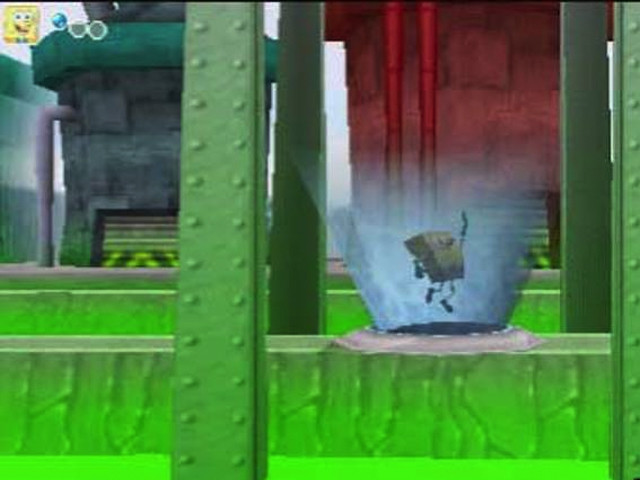This screenshot from a cartoony, animated video game prominently features SpongeBob SquarePants, recognizable by his yellow sponge appearance with arms and hands. SpongeBob is depicted standing on green metallic infrastructure that suggests a setting within a nuclear plant. The environment is further accentuated by various elements: a purple-blue glowing orb to the right side of the image, big red structures equipped with garage doors, and another similarly styled silo structure. In the top left corner, there's a SpongeBob SquarePants logo accompanied by indicators that seem to display his health or life status.